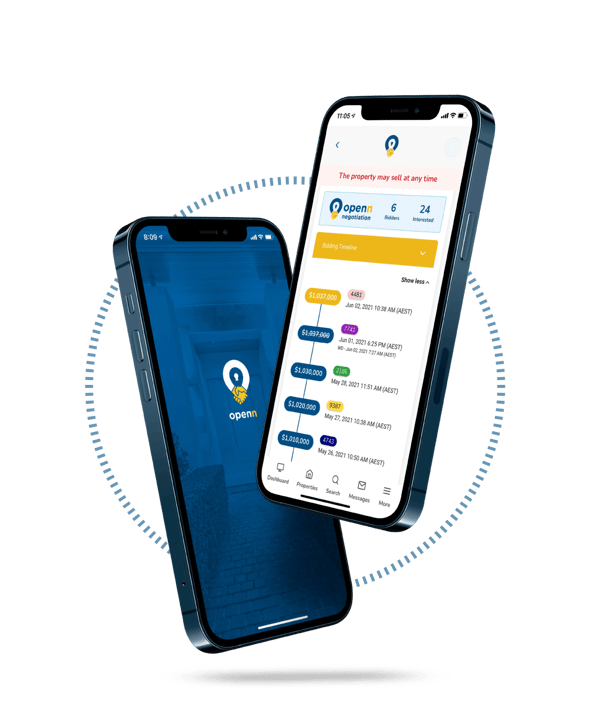The image features two smartphones set against a background comprised of a large blue circle made up of small blue lines forming a cohesive circular design. Within this circle are the two prominently displayed smartphones.

The first smartphone showcases a home screen with a blue wallpaper. The visible background image includes a ground composed of brickwork and what appears to be a white door. On the smartphone's screen, there is a prominent white circle with the word "Open" displayed underneath.

The second smartphone's screen is open to a website page. At the top of the webpage, a red notification reads, "The property may sell at any time." Adjacent to the brand name "Open" (spelled O-P-E-N-N), there are numbers "6" and "24." Further down the screen, an orange banner is visible, completing the display of information on this fictional website.

Together, these elements create a visually coherent and informative representation, placing emphasis on the smartphones and the user interfaces they display.